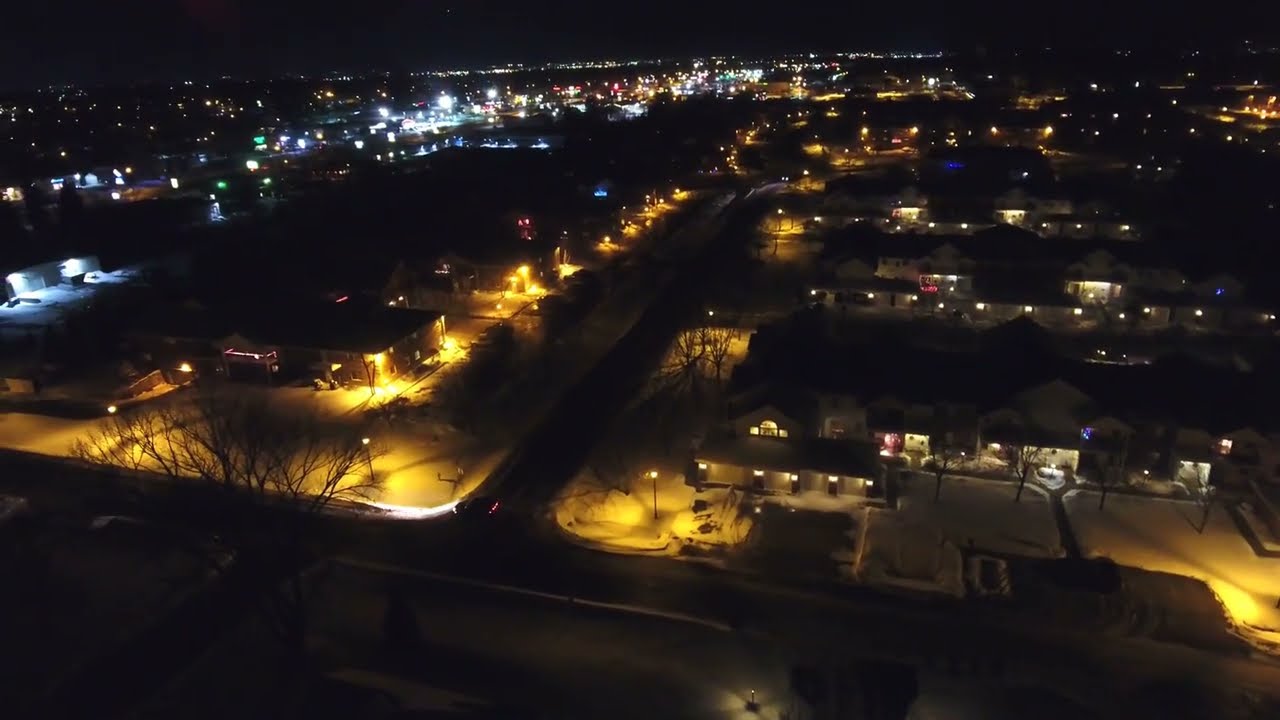This aerial, horizontal image captures an urban area at night, showcasing a stark contrast between a largely dark foreground, possibly a park, and a brightly lit residential neighborhood. Running through the middle of the image is a prominently lit street, flanked by yellow streetlights, leading into blocks of houses that appear to be part of a suburban area. The homes, particularly on the right, are large and well-lit, resembling mansions with glowing lights on their fronts and yellow streetlights lining the roads. On the left side of the image, the urban landscape transitions to what appears to be a commercial or city area, distinguished by white streetlights and building lights, including possible stores and busy roads. The background further merges into the broader cityscape, with varying spots of yellow and white lights. The sky is a deep black, emphasizing the nighttime setting and the artificial illumination that defines the scene. A hint of snow on the ground adds to the overall atmosphere, reflecting the streetlights and contributing to the image's detailed night-time tableau.